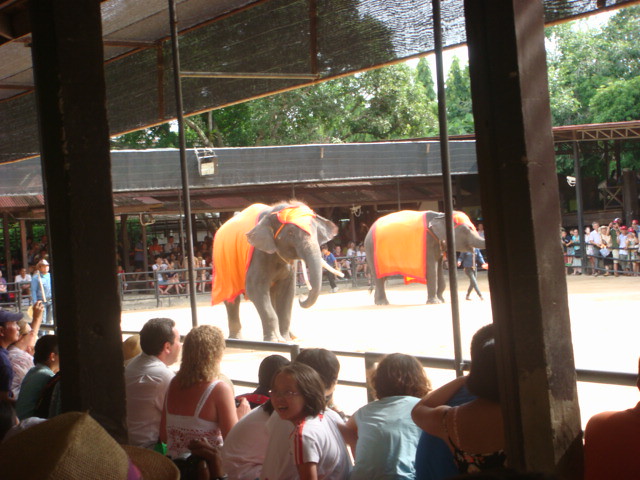The photograph captures an outdoor scene at a zoo or nature park where an elephant show is taking place. In the background, a lush canopy of green trees is visible, framing an open-air arena. This enclosure, which has a roof wrapping around it, houses spectators seated on benches and bleachers, attentively watching the performance. Inside the sandy-floored arena, two elephants, each adorned with an orange cloth draped over their backs and a matching headdress, are accompanied by their trainers. A railing separates the audience from the elephants, ensuring safety. The sunlight bathes the scene, highlighting the elephants and creating a vivid daytime atmosphere. The image, captured with an amateur camera, showcases a lively moment filled with natural beauty and human-animal interaction.